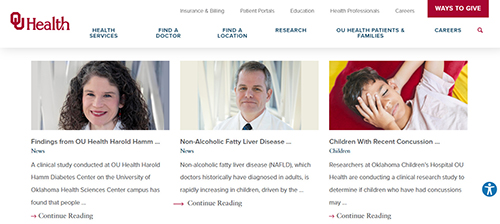The image showcases a webpage with a pristine white background. In the upper left corner, the words "OU Health" are prominently displayed in bold red letters. To the right of this, there are five menu options in gray text, which are unfortunately too small to decipher. Directly next to these options is a red box featuring the text "Ways to Give" in white font.

Below this top menu, there are another six menu options in blue text, again too small to be clearly read. On the far right of this section, there's an icon of a magnifying glass, suggesting the presence of a search function.

The main section of the webpage features three tiles arranged side by side. The first tile on the left displays an image of a woman with brown hair wearing red lipstick. The middle tile shows a man dressed in a white shirt and tie. The final tile on the right depicts a child lying down with one hand covering his face.

Each of these tiles has a title and a brief description underneath, although the text is quite small. The title under the third tile reads "Children with Recent Concussion." The middle tile is titled "Non-Alcoholic Fatty Liver Disease." The title under the first tile references OU Health, but the text is too minute to fully discern. Beneath each title, there are a few lines of descriptive text, though the small font size poses a challenge for readability.